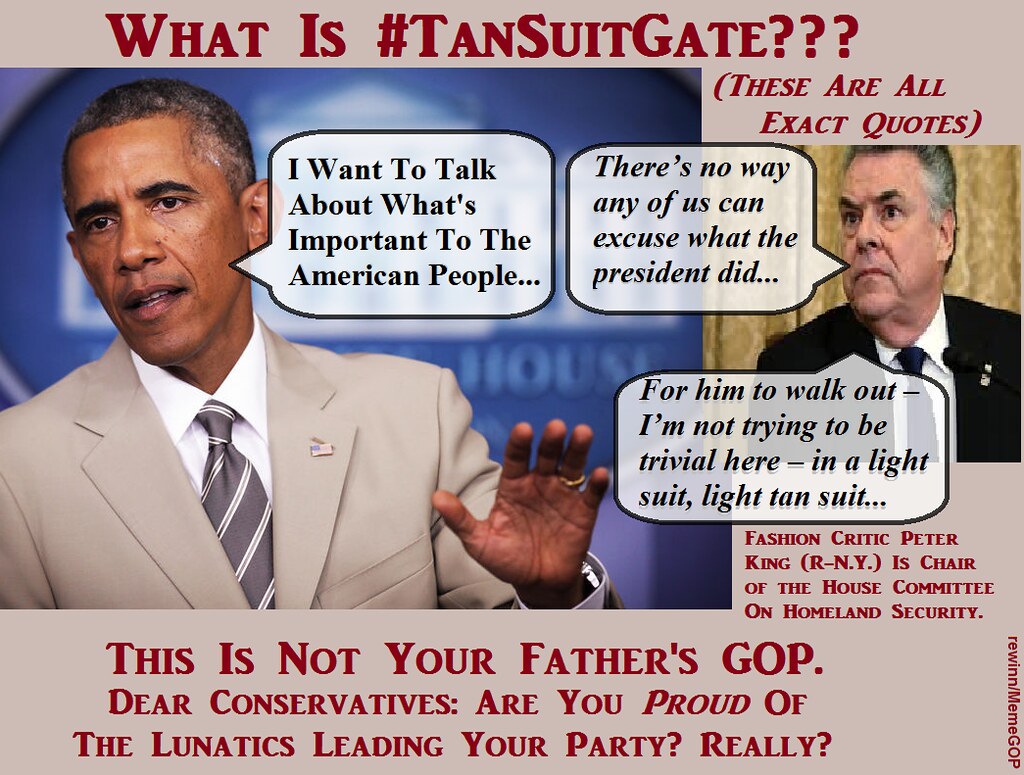The image is a politically charged meme featuring a split-screen composition. On the left, President Obama is depicted mid-speech, wearing a cream-colored suit, gray striped tie, and white shirt, with an American flag pin on his lapel. His cartoon speech bubble reads, "I want to talk about what's important to the American people." On the right, in a smaller square, an older gentleman in a dark suit, identified as Representative Peter King from New York, looks serious and quizzical. His caption states, "There is no way any of us can excuse what the president did. For him to walk out in a light suit, a light tan suit. I'm not trying to be trivial here." Above the images, the text reads, "What is #TanSuitGate???" in red, questioning the controversy surrounding Obama's suit choice. At the bottom, more red text declares, "This is not your father's GOP, dear conservatives. Are you proud of the lunatics leading your party? Really?" The overall design critiques the reaction to Obama's unconventional suit choice and questions contemporary conservative leadership.